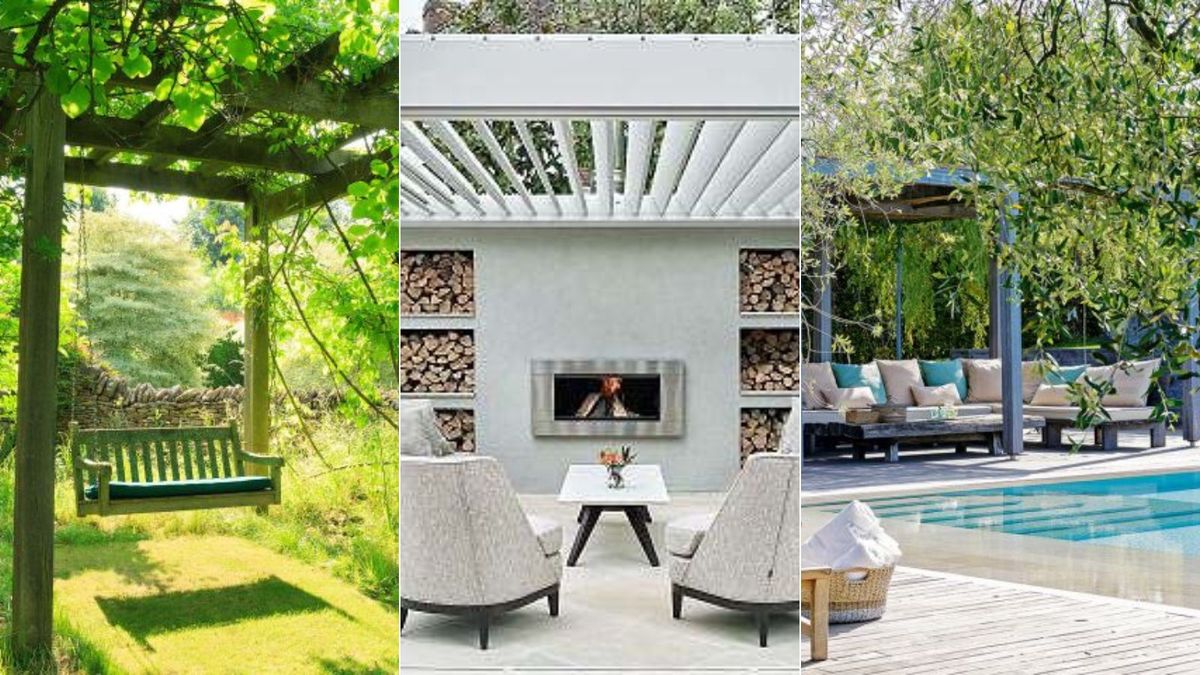The image consists of three outdoor scenes captured in daylight. 

The left scene features a verdant outdoor setting with a green arbor overhead, thickly draped in vines and foliage casting dappled sunlight. Under the arbor stands a green wooden swing with a blue cushion, above a patch of short, light green grass. The scenery around it is lush and overflowing with various shades of green.

The center scene showcases an open-space patio under a white arbor with slatted roofing, allowing glimpses of the sky. A fireplace is centrally featured, surrounded by organized stacks of chopped wood in six rectangular compartments on either side. Two white chairs with beige patterns face the fireplace, which is encased in a sleek silver rectangle with a black interior. A white table with wooden legs stands in the middle, adorned with flowers.

The right scene presents a tranquil poolside area under a blue, vine-covered arbor. There's a large outdoor sofa with beige and blue cushions positioned adjacent to the pool, complemented by a basket of blue towels nearby. A marble-tiled surface edges the pool, while stairs lead into the cyan-hued water. Overhanging tree branches provide shaded relief, adding to the serene atmosphere.

Each scene illustrates a different facet of outdoor leisure, collectively emphasizing lush greenery, thoughtful design, and inviting comfort.